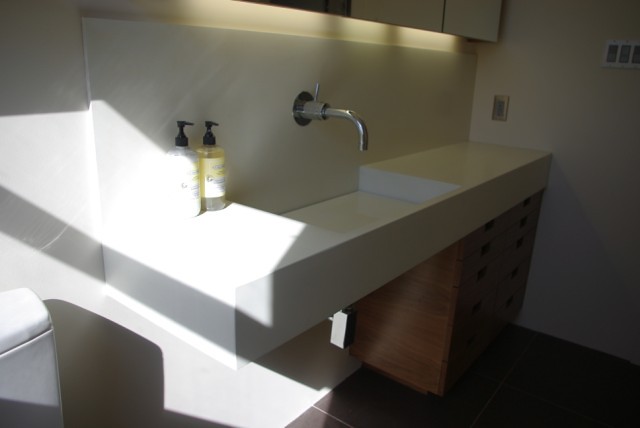In this image, we see the corner of a bathroom. At the top, a white cupboard is partially visible. Below the cupboard, there is a white ceramic hand-washing sink. The sink is installed against both the back wall and an adjacent wall, firmly situated in the corner. Beneath the sink, there are wooden drawers adding a touch of contrast to the setup. On the right side of the sink, two bottles of hand soap are neatly placed. To the left of the sink, the edge of a toilet is visible, completing the functional layout of this bathroom corner.